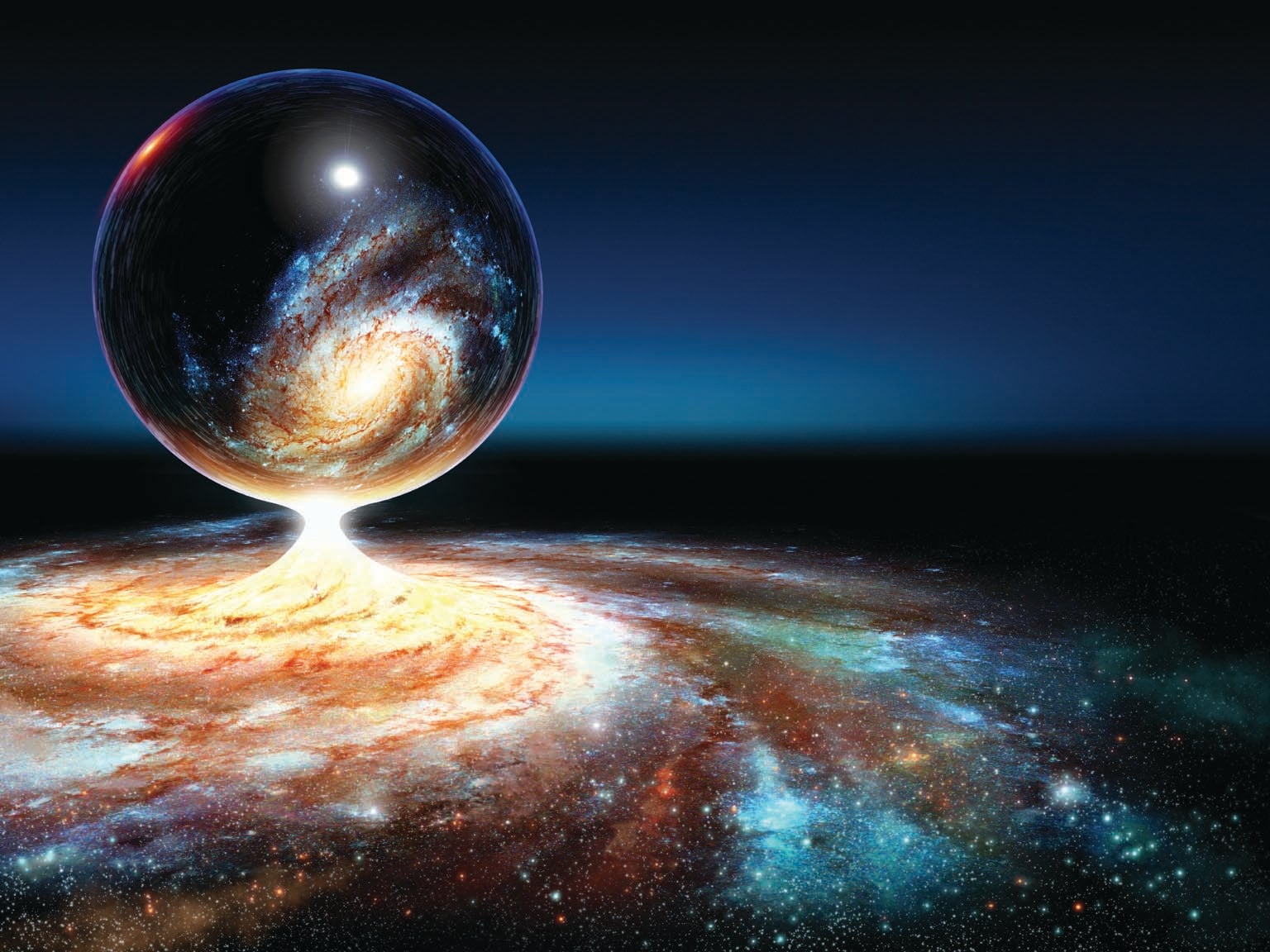This detailed illustration portrays a mesmerizing outer space scene. The top half of the background is a gradation from dark blue to a slightly lighter blue, creating a deep, cosmic ambiance. Dominating the upper left-hand corner is a shiny, black reflective sphere. Inside this sphere, there's a bright yellow swirl that resembles either a nebula or a galaxy, encircled by swirling cloud-like formations in colors of red, light blue, and darker blue.

Located below this reflective sphere is an expansive, vivid galaxy scene. This galaxy is characterized by a prominent orange swirl on the left side, extending upward in a conical shape, seemingly touching the bottom of the sphere. The galaxy spans the lower half of the image with vibrant red and yellow swirling areas, blending into regions of blues, oranges, and countless small white star-like lights scattered throughout. The lower point of the galaxy transitions seamlessly into the vast field of stars and nebulous regions, highlighting the wonder and depth of the universe.